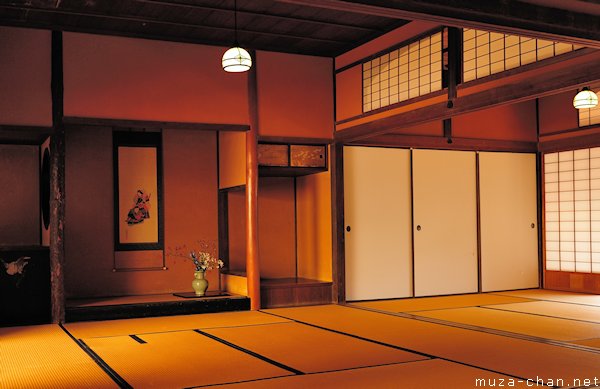This photograph captures the serene interior of a Japanese-style house, characterized by its traditional design elements and muted color palette of light orange, cream, black, and dark brown. The floor features light orange tatami mats bordered in black, adding to the authentic Japanese aesthetic. On the right side, three light cream sliding doors with small recessed circular areas stand closed, alongside glazed windows. The room is softly illuminated by two white overhead light fixtures. On the left, a green vase with flowers sits on the ground, and an Asian-inspired scroll or tapestry hangs on the wall, adding to the tranquil ambiance. The walls are crafted from a beautiful brown wood, enhancing the natural feel of the space. The only text visible in the bottom right corner of the image reads "moozachand.net," leaving the function of the room—whether a spa, boutique, or home—open to interpretation.